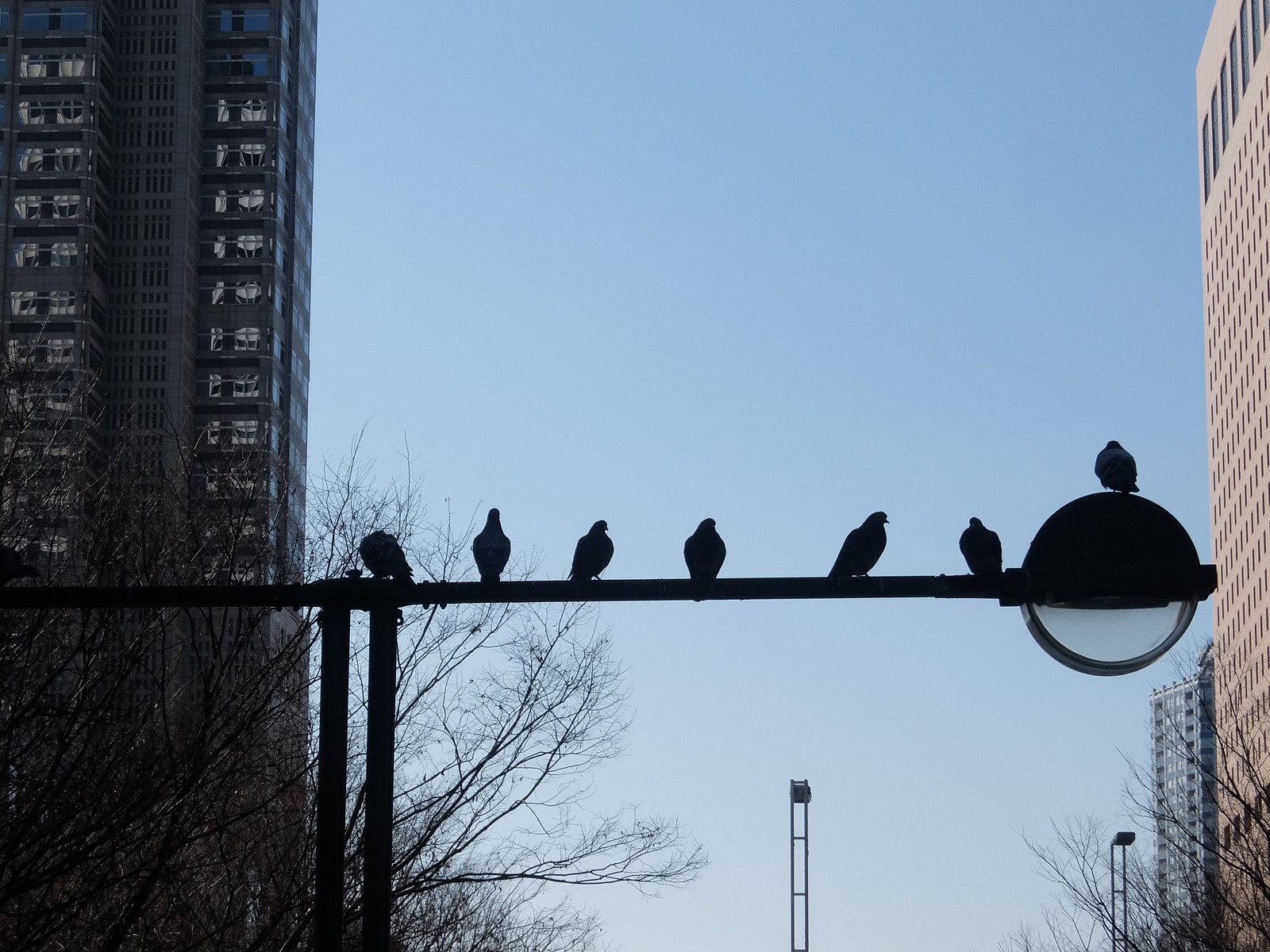The photograph captures an urban scene with prominent buildings on both sides—on the left, a towering black-gray building, and on the right, a tall tan structure, likely skyscrapers. Dominating the foreground is a modern streetlight with a birds-eye-view perspective. The streetlight features a horizontal metal rod extending across much of the frame, supported by vertical pipes. Seven pigeons are perched along this rod, with six clustered together on the horizontal bar and one singular pigeon atop the circular streetlight head. The streetlight itself is designed with a metallic top and a U-shaped glass bottom, creating a distinctive look. The background showcases a clear, cloudless sky, indicating a bright, sunny day, contrasting with the dormant, leafless trees scattered across the scene, suggesting it is winter. The clear focus and detailed elements create a vivid depiction of a bustling, yet serene urban landscape.